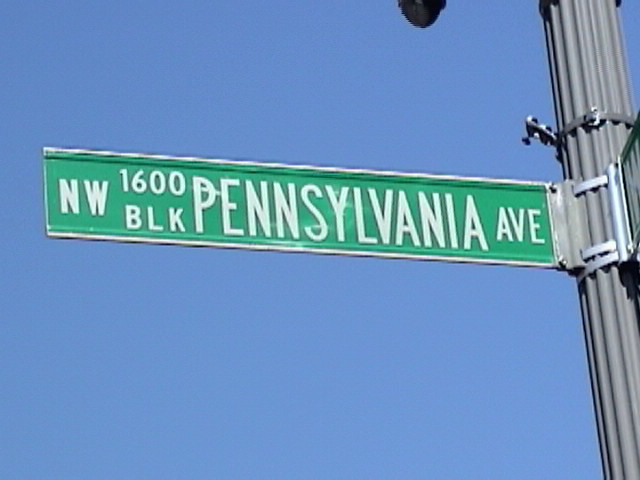Under a completely clear, medium blue sky, a street sign attached to a thick, gray, vertically ribbed pole stands prominently. The metal-mounted sign at the top of the pole is a long, narrow rectangle with a green background and white, capitalized lettering. It reads "NW 1600" at the top and "BLK" underneath, with the word "PENNSYLVANIA" spelled out in large, bold letters across the middle, followed by "AVE" at the bottom. A bracket on the pole holds the edge of another sign extending at a 45-degree angle, although the sign's text is not visible in this image.